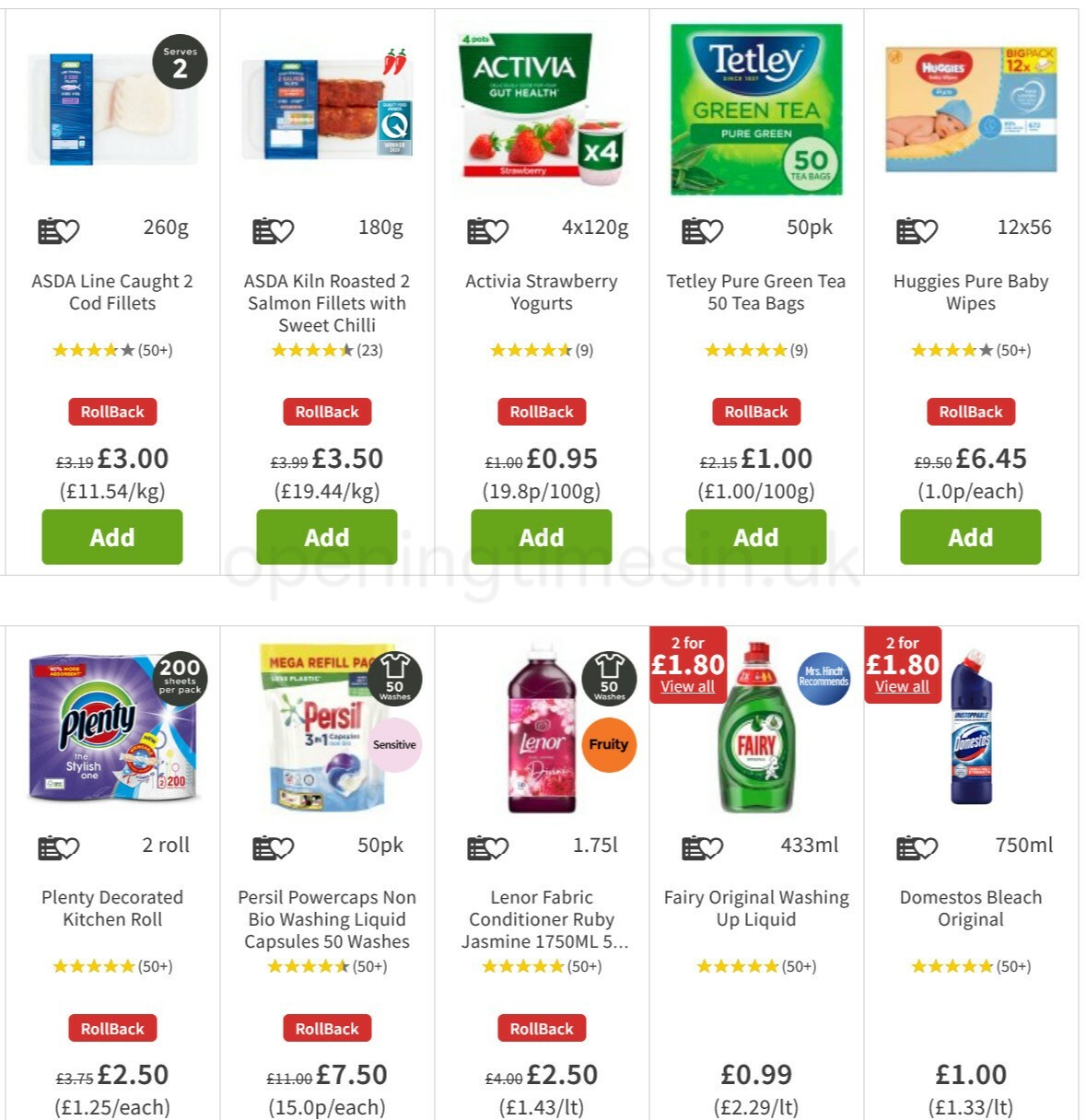The image is a cropped screenshot displaying a series of digital advertisements, organized into two rows of five ads each. Each ad is formatted as a vertical rectangle. At the top of each ad, there are images of the featured items, accompanied by their names, reviews, and ratings. A red button labeled "Rollback" indicates a price reduction, followed by the price of the item. At the bottom, a green button with "Add" in white text allows users to add the item to their cart.

### Top Row (Left to Right):
1. **ASDA Line Caught 2 Cod Fillets** - Priced at £3.00
2. **ASDA Kiln Roasted 2 Salmon Fillets with Sweet Chili** - Priced at £3.50
3. **Activia Strawberry Yogurts** - Priced at £0.95
4. **Tetley Pure Green Tea 50 Tea Bags** - Priced at £1.00
5. **Huggies Pure Baby Wipes** - Priced at £6.45

### Bottom Row (Left to Right):
1. **Plenty Decorated Kitchen Roll (2 for 2)** - Priced at £2.50
2. **Persil Power Caps Non-Bio Washing Liquid Capsules (50 washes)** - Priced at £7.50
3. **Lenore Fabric Conditioner Ruby Jasmine (1750 milliliters)** - Priced at £2.50
4. **Fairy Original Washing Up Liquid** - Priced at £0.99
5. **Domestos Bleach Original** - Priced at £1.00